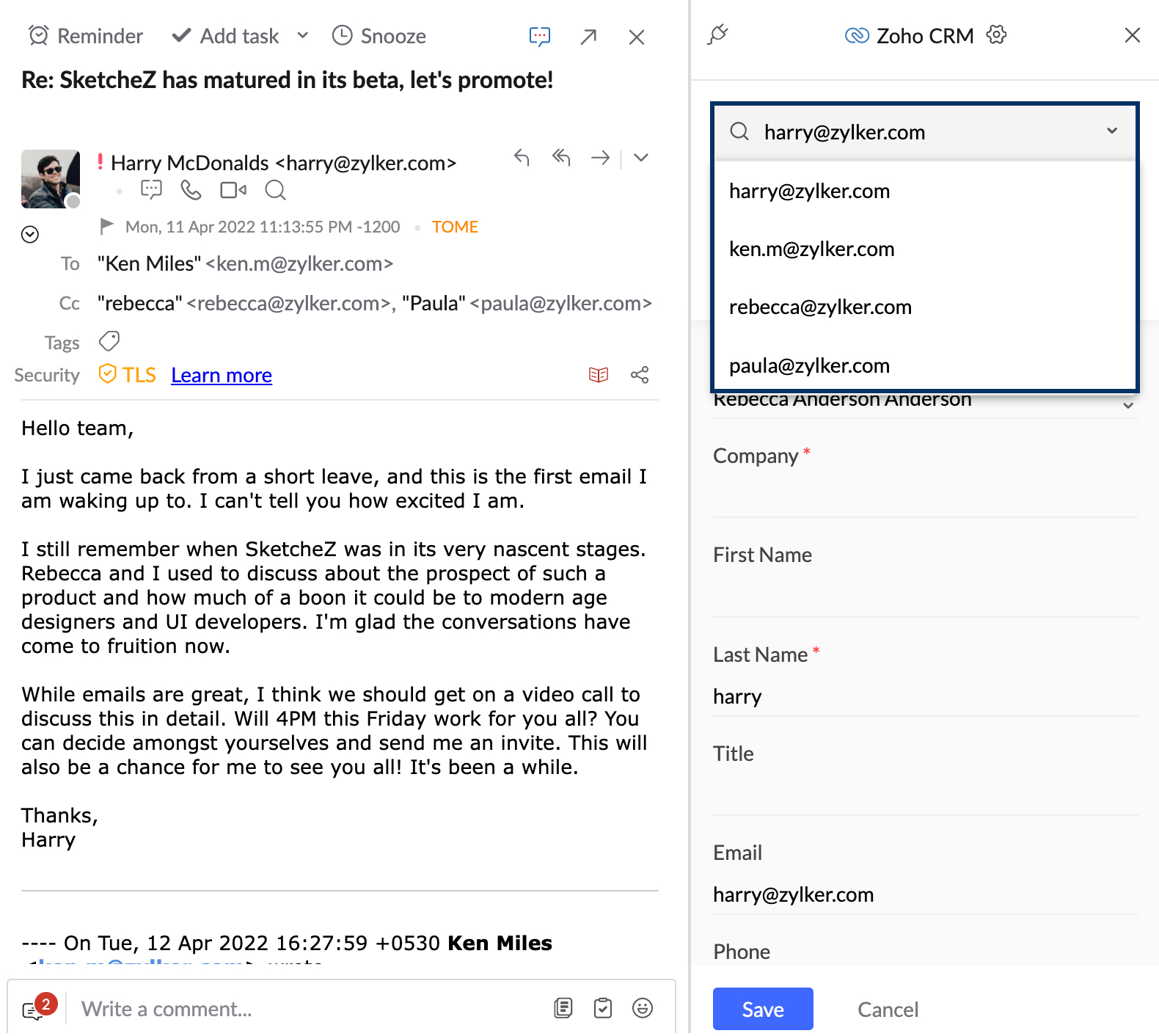**Detailed Descriptive Caption for Screenshot of Email Interface**

The image is a detailed screenshot of an email interface with multiple functionalities visible. On the top left-hand side, there are options labeled "Reminder," "Add Task," and "Snooze." Below these options, there are icons representing a text chat box, an arrow, and an "X". 

The email subject reads, "RE: Sketches has matured in its beta, let's promote," and is from Harry McDonald (harry@zylker.com). The email was sent on Monday, April 11, 2022, at 11:13:55 PM. It is addressed to Ken Miles (kenm@zylker.com) with Rebecca (rebecca@zylker.com) and Paula in CC.

The body of the email begins with a friendly greeting: "Hey, team," and Harry mentions his recent return from a short leave. He expresses excitement upon seeing the email about the development of "Sketches," reminiscing about the early discussions with Rebecca regarding the product's potential impact on designers and UI developers. Harry is pleased that those early conversations have now borne fruit. He suggests that the team should have a video call to discuss this further and proposes Friday at 4 PM for the meeting. He also mentions his eagerness to see everyone, as it has been a while since they last met. The email concludes with a thanks from Harry.

On the right-hand side of the interface, there is a section indicating "Zoho CRM." This section includes a gear icon for settings, a search bar for typing in email addresses to look up contacts, and a display of contact information beneath the search bar.

**End of Caption**